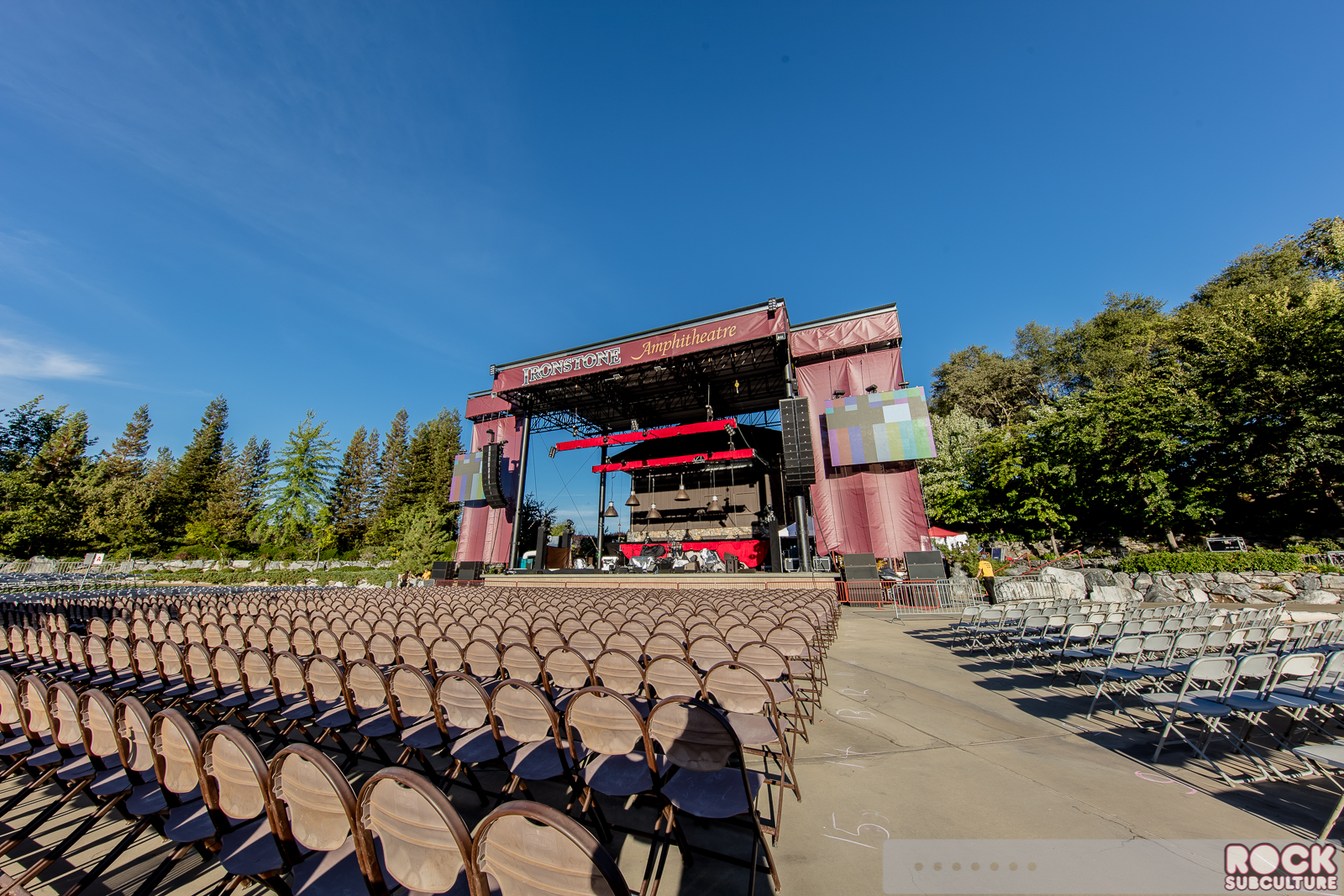The image is a vibrant color photograph depicting an outdoor amphitheater on a bright, sunny day with a clear blue sky. The stage, primarily red in color with some tan accents, is situated centrally within the scene and flanked by lush green trees, indicating a late spring to early fall season. The stage features two sizable TVs, one on either side. Rows of chairs are neatly arranged in front of the stage. The central rows consist of larger chairs with circular backs made of light brown material and dark brown frames, while the side sections are populated by standard gray metal folding chairs. Musical instruments are positioned on the stage, hinting at an upcoming performance. Sparse figures can be seen in the distance, presumably setting up for the event. On the bottom right of the image, the number "15" is visible on the sidewalk, and a strip of text reads "Rock Subculture."